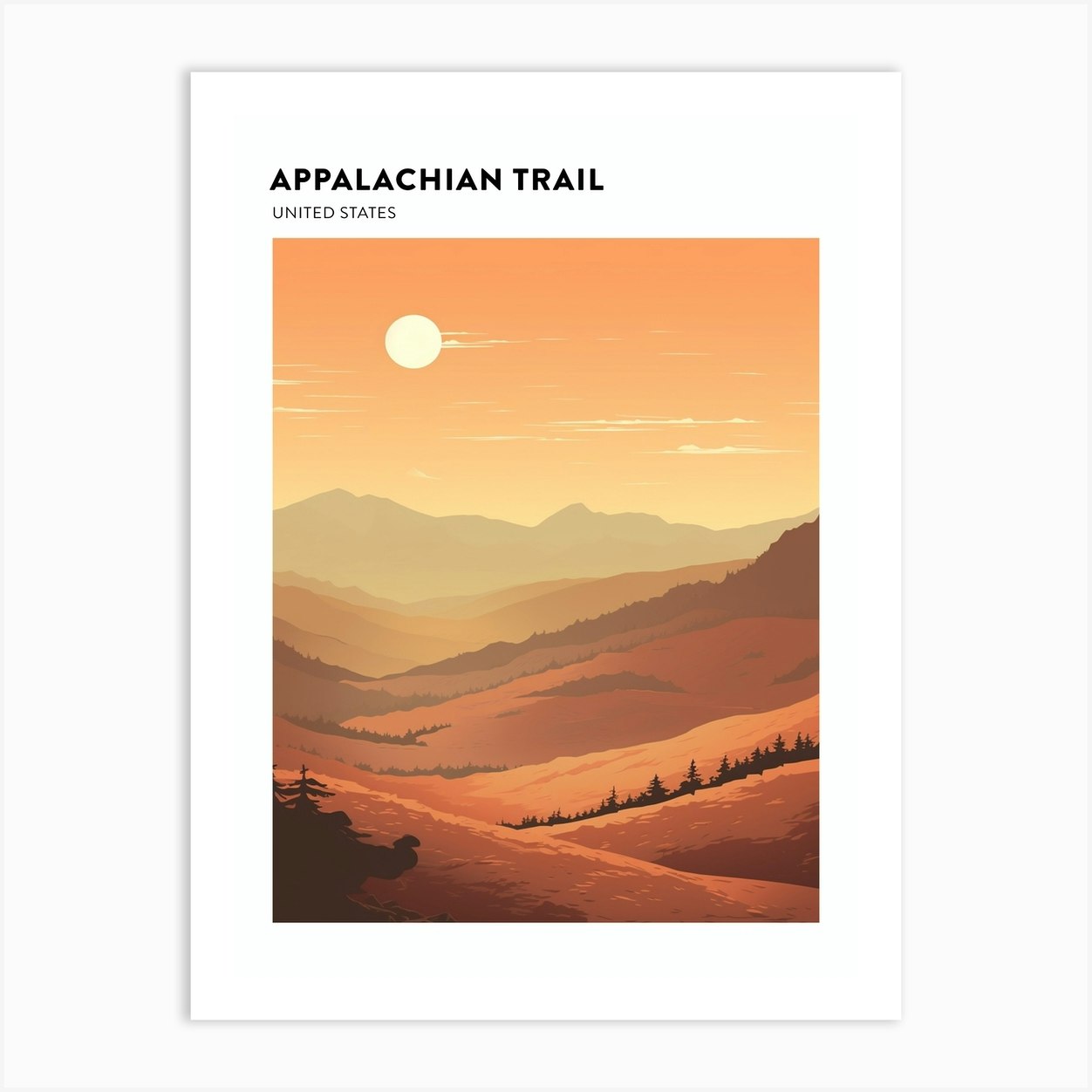The image on a sheet of plain white paper prominently features the bold, black, all-capitalized title "APPALACHIAN TRAIL" at the top, followed by the smaller text "United States." Below the text is a vibrant image featuring a dynamic range of colors from reds and yellows to darker browns. A bright, circular sun sits high in the sky, accompanied by faintly colored mountains in the background that progressively darken as they approach the viewer. The foreground includes very dark trees situated on smaller hills and some darker markings suggesting foliage. The hills gradually become larger towards the back of the picture, with mountain ranges in the distance depicted in darker tones, contrasting with lighter brown mountains highlighted with some dark shading. The image is reminiscent of a book or poster, bordered by a thick white frame, and even includes clouds with a light yellow tint, adding depth to the atmospheric landscape.